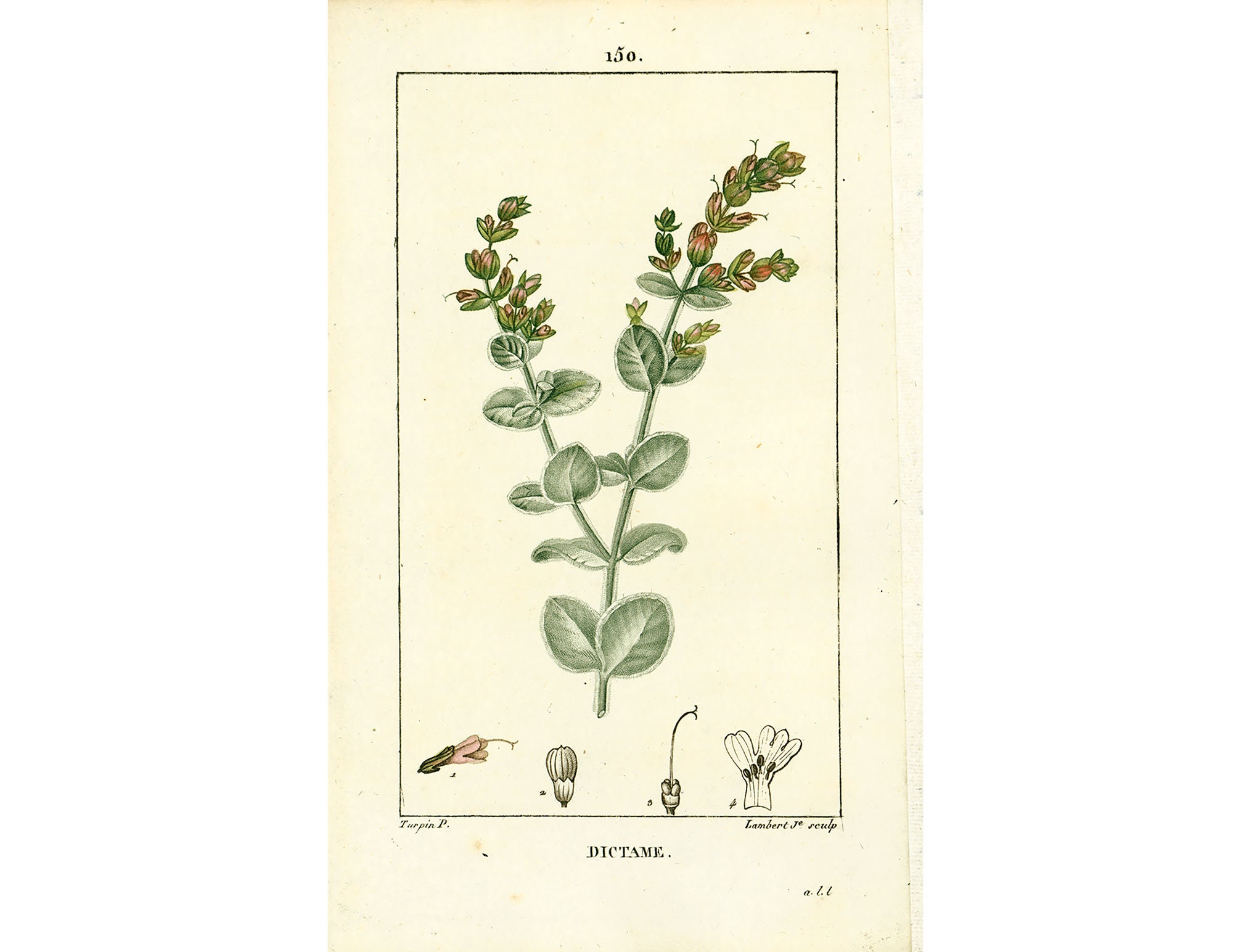This image is a detailed botanical illustration of a plant, seemingly hand-painted on a beige, cream-colored background. The central figure is framed with a thin black rectangular border. At the top of the illustration, the number 150 is prominently displayed. The main plant within the border features two long stems with multiple layers of large green leaves branching out symmetrically. The taller stem, situated on the right side, showcases gold buds sprouting from it, while the shorter left stem mirrors this growth pattern with similarly grouped leaves and buds. At the top of these stems, delicate pink flowers can be seen. 

Below the central plant, there are smaller, detailed illustrations depicting different parts of the plant labeled A, B, and C, but without a legend for reference. Additionally, the bottom of the image is marked with the text "Dictame," and further annotated with signatures, "Turpin P." on the left side and "Lambert J. Sculpe" on the bottom right. These annotations suggest the collaborative effort of the illustrators. Overall, this artwork likely represents various stages of the plant's growth, capturing its detailed morphology in a style reminiscent of traditional botanical sketches typically found in historical manuscripts or botanical books.